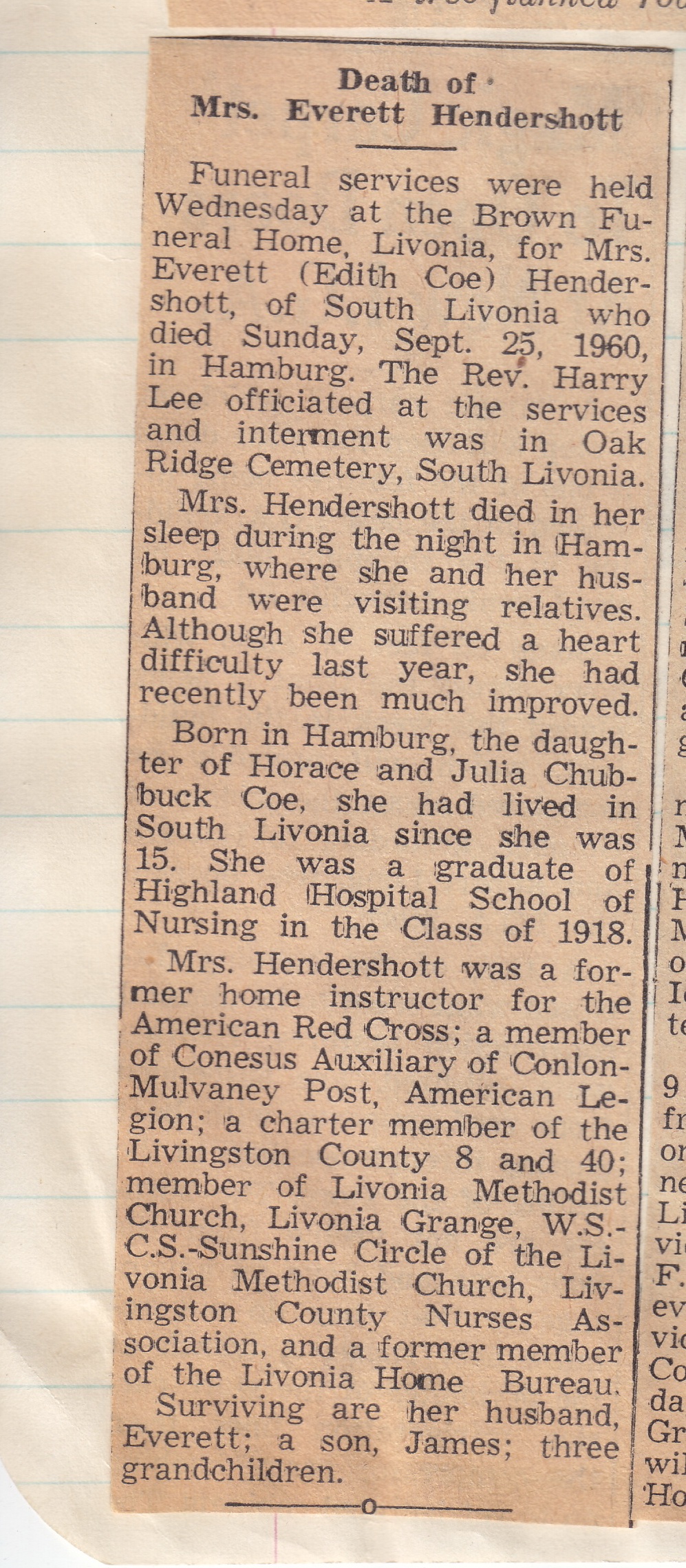The image is a vertically aligned rectangular picture of a clipped newspaper obituary, placed on a white sheet of notebook paper marked with horizontal blue lines. The aged, beige-toned paper reveals its old nature. At the top, the bold black text reads "Death of Mrs. Everett Hendershot." The obituary mentions that funeral services were held on Wednesday at the Brown Funeral Home in Livonia for Mrs. Everett (Edith Coe) Hendershot of South Livonia, who passed away on Sunday, September 25th, 1960, in Hamburg. The Reverend Harry Lee officiated at the services, and the interment was in Oak Ridge Cemetery, South Livonia. The text continues, stating that Mrs. Hendershot died in her sleep during the night in Hamburg while visiting relatives with her husband, despite having suffered a heart difficulty the previous year, from which she had shown significant improvement. 

Born in Hamburg to Horace and Julia Chubbuck Coe, Mrs. Hendershot moved to South Livonia at the age of 15 and graduated from Highland Hospital School of Nursing in the class of 1918. She had been a former home instructor for the American Red Cross, a member of the Constance Auxiliary of Conlon-Mulvaney Post American Legion, a charter member of the Livingston County 8 and 40, a member of Livonia Methodist Church and its WSCS Sunshine Circle, Livonia Grange, and the Livingston County Nurses Association. She was also a former member of the Livonia Home Bureau. Surviving her are her husband, Everett, a son named James, and three grandchildren.